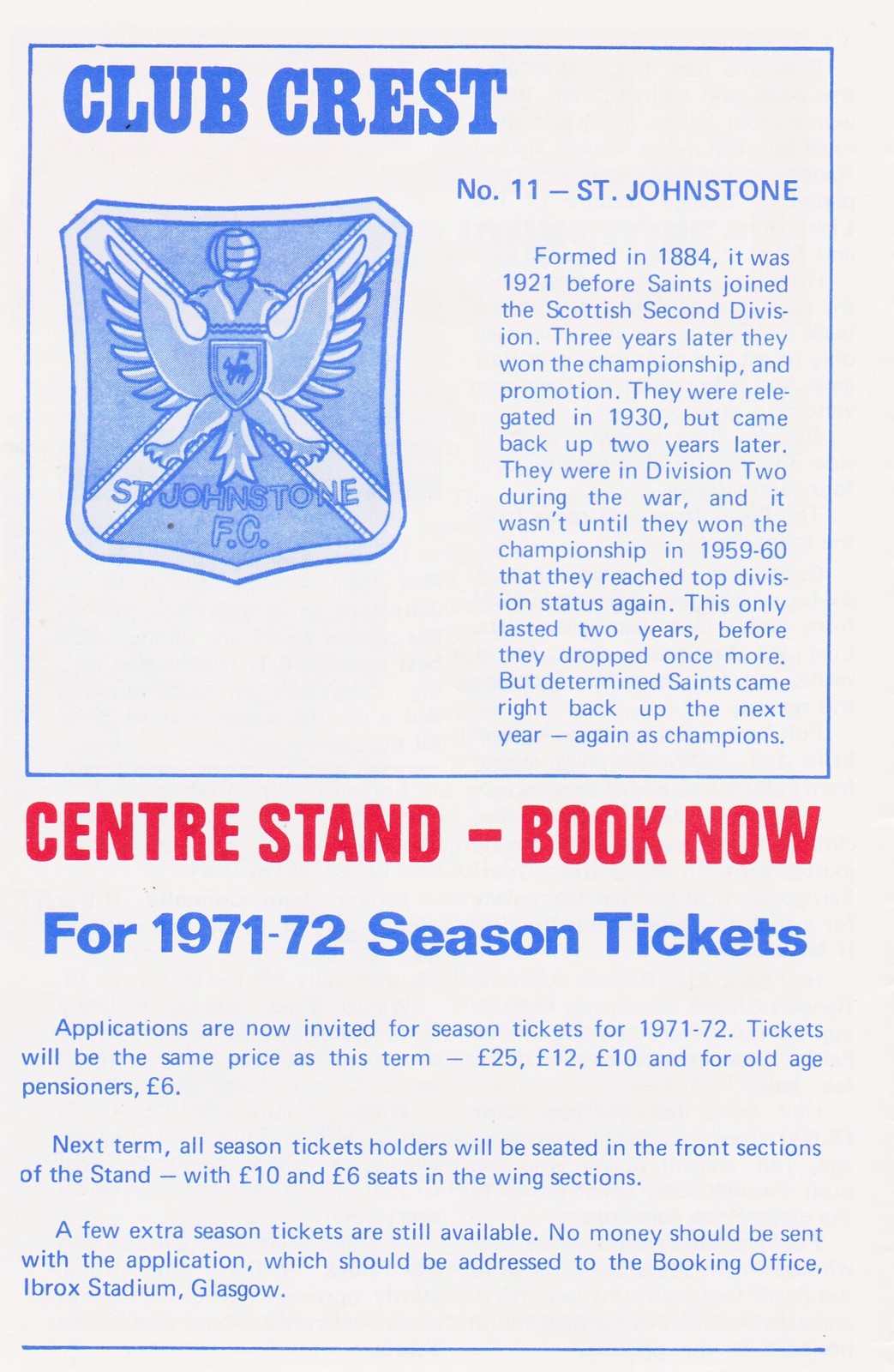The image is a promotional poster for St. Johnstone FC's 1971-72 season tickets. The background is white and the poster is displayed in a vertical rectangle format. In the top half, there is an almost-square blue border. Inside this border, the background remains white. The upper left corner of the blue frame features bold blue text reading "Club Crest." Just below and to the right of this, smaller text is right-justified, stating "NUMBER 11 ST. JOHNSTONE" in all caps. 

Beneath this text, a paragraph of blue text is fully justified but too small to read clearly. To the left of this paragraph, there is a blue and white crest depicted as a blue, angled-cornered shield. The shield showcases a design of crossed bats or clubs with a pair of wings and a helmeted player in the middle. At the bottom of the shield, in slightly darker blue text, are the words "St. Johnstone."

In the lower half of the image, below the blue outlined square, bold red, all-caps text reads "CENTRE STAND - BOOK NOW." Following this, a line of smaller blue text announces "FOR 1971-72 SEASON TICKETS." 

Further down, three paragraphs of blue text detail the ticketing information:
1. "Applications are now invited for season tickets for 1971-72. Tickets will be the same price as this term - £25, £12, £10. For old age pensioners, £6."
2. "Next term, all season ticket holders will be seated in the front sections of the stand, with £10 and £6 seats in the wing sections."
3. "A few extra season tickets are still available. No money should be sent with the application, which should be addressed to the Booking Office, Ibrox Stadium, Glasgow."

A horizontal blue line marks the bottom of the image.